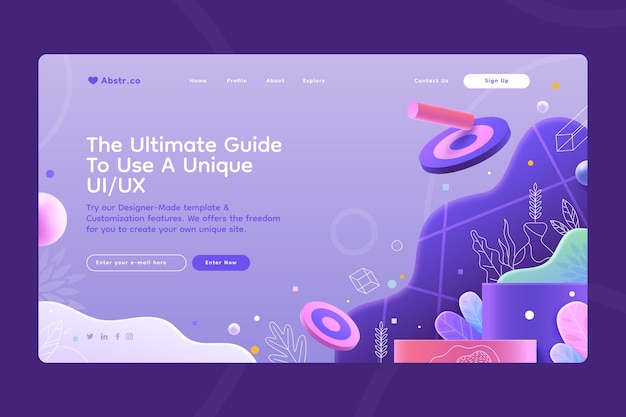The image is a screenshot of a website featuring a dark purple border that surrounds the main content. Within the screenshot, the central website displays a text-centric page with a patterned background consisting of white geometric cubes, leaf outlines, and colorful target shapes.

In the top left corner of the screenshot, a purple heart icon accompanies text reading "abstr.co." The navigation bar centered at the top enumerates the following links in white text: "Home," "Profile," "About," "Explore," and "Contact Us," with a "Sign Up" button in purple text inside a white pill-shaped button located at the far right.

To the left of the screenshot's main area, a bold white heading declares, "The Ultimate Guide to Using a Unique UI/UX." Below this heading, purple text encourages users to "Try our designer-made template and customization features. We offer the freedom for you to create your own unique site." Further down, white text prompts users to "Enter your email here," accompanied by a boxed section marked "Enter Now." The bottom segment of this sidebar includes social media icons for Twitter, LinkedIn, Facebook, and Instagram.